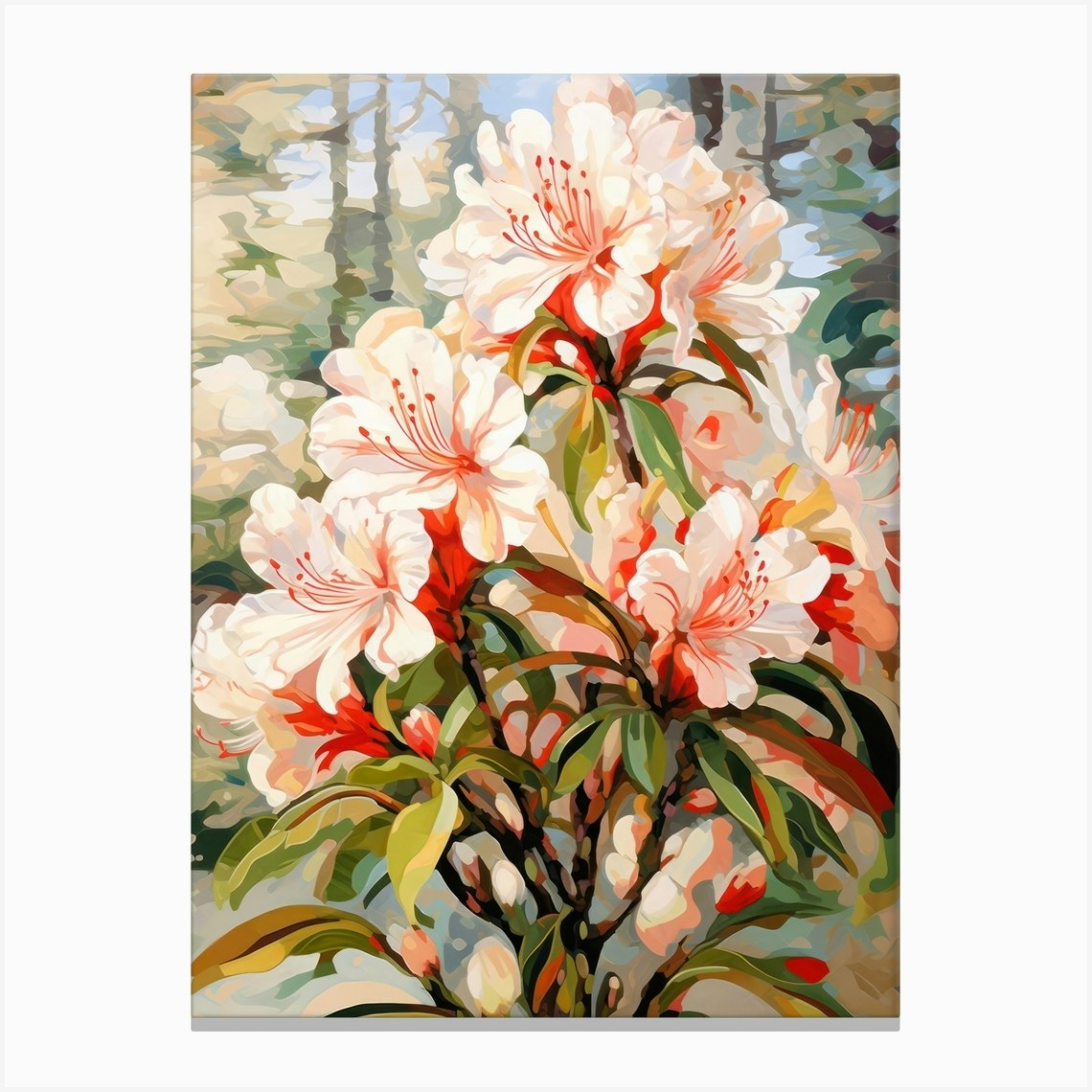This detailed painting showcases a stunning arrangement of flowers with intricate details and a vibrant background. Central to the composition are several blooms with layers of white petals, each accented by a bright orange at their base. These exquisite flowers feature delicate, thin green leaves and long stems, with prominent orange protrusions with a tiny ball at the tip emerging from their centers. Surrounding the flowers, the background reveals a serene landscape of tall trees, painted against a blue sky, hinting at a forest setting. This almost watercolor-like scenery includes varying shades of green for the leaves and tree trunks in a dark gray. The atmosphere seamlessly transitions to a potentially ambiguous ground or water at the bottom, depicted in gray tones and showing the bases of the trees. This harmonious blend of elements creates a captivating and tranquil scene that beautifully balances the foreground's floral details with the gentle blur of nature in the background.